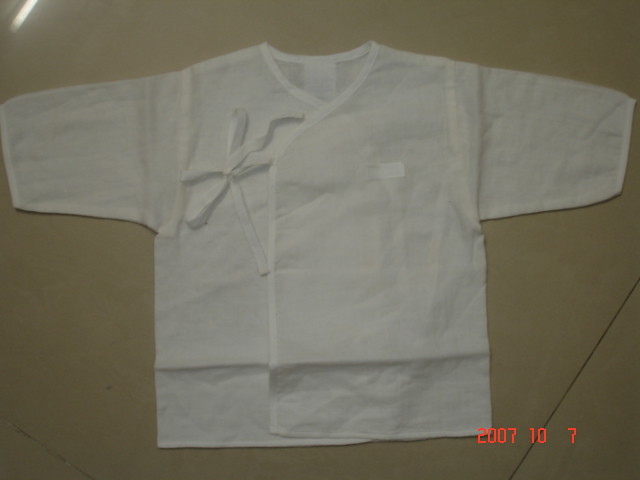An overhead photograph captures a white scrub top laid flat against a shiny gray, possibly reflective surface. The scrub's short sleeves are spread out to the sides. The top features a wrap-style design with two front panels that overlap, secured by ties resembling shoelaces on the upper left side. This V-neck garment, appearing as though it would reach just to the waistline, showcases its lightweight material vividly against the subdued background. In the bottom right corner, red lettering indicates the date the picture was taken: October 7th, 2007.